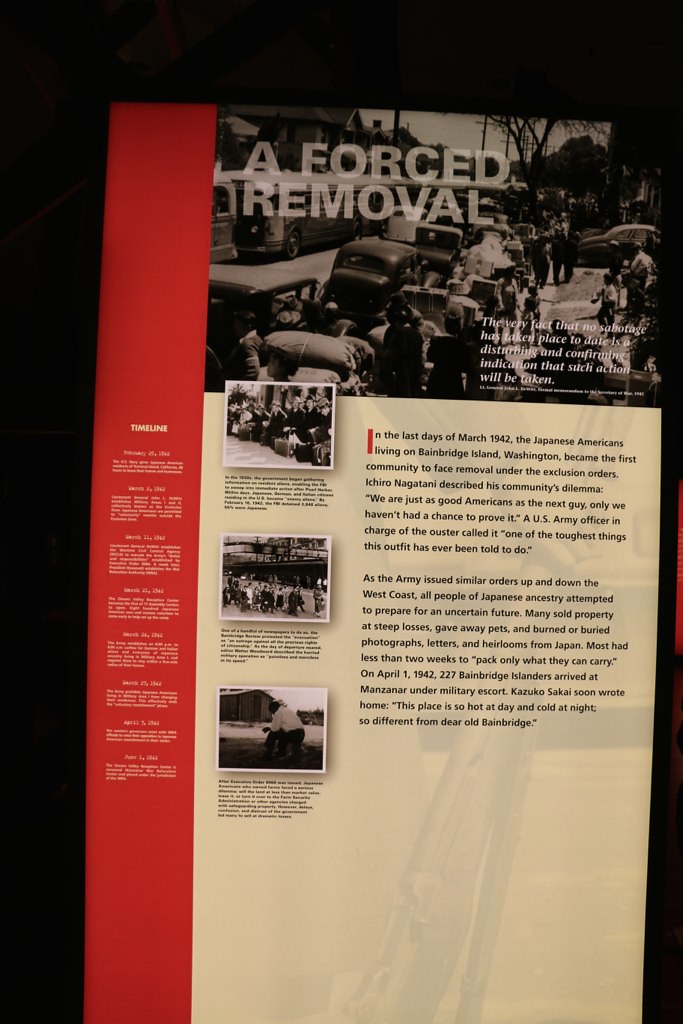The image appears to be from a military museum exhibit, featuring a large rectangular sign with a black background and a red strip on the left labeled "Timeline," listing eight dates with corresponding synopses. The top of the exhibit showcases an old black-and-white photograph of numerous cars lined up on a street, depicting people leaving under duress. In white letters atop this image, it states "A Forced Removal," signaling the nature of the scene. To the bottom right of the photograph, a caption reads: "The very fact that no sabotage has taken place to date is a disturbing and confirming indication that such action will be taken." Adjacent to these elements, there's an extensive white area filled with black text that details the historical context. The text begins: "In the last days of March 1942, the Japanese Americans living on Bainbridge Island, Washington, became the first community to face removal under the exclusion orders." It includes a poignant quote from Ichiro Nagatani, who lamented, "We are just as good Americans as the next guy, only we haven't had a chance to prove it." Additionally, it cites a U.S. Army officer in charge of the operation, remarking it was "one of the toughest things this office has ever been told to do." The display evokes the tragic displacement of Japanese Americans during World War II.